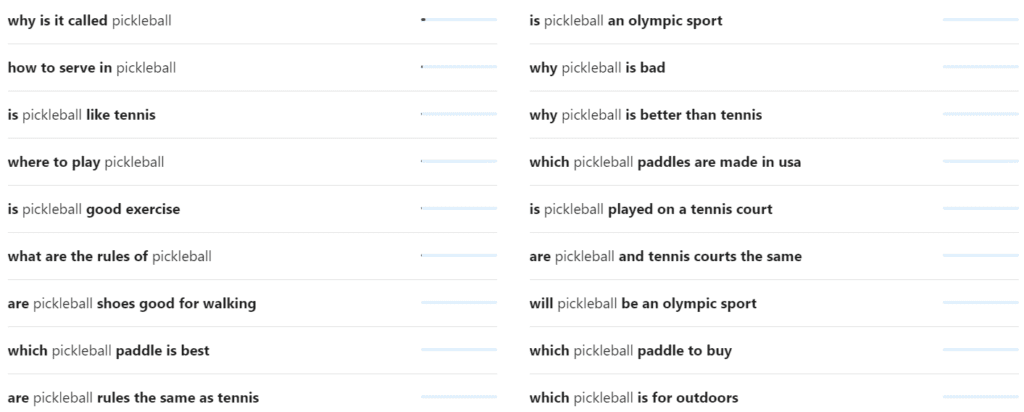This image depicts a search results page from an unspecified website, possibly Google or Wikipedia, based on the layout and content. The query appears to be about "pickleball." The page is populated with various collapsible sections containing frequently asked questions (FAQs) related to the sport. Questions include: "Why is it called pickleball?", "How to serve in pickleball?", "Is pickleball like tennis?", "Where to play pickleball?", "Is pickleball good exercise?", "What are the rules of pickleball?", "Are pickleball shoes good for walking?", "Which pickleball paddle is best?", "Are pickleball rules the same as tennis?", "Is pickleball an Olympic sport?", "Why is pickleball bad?", "Why is pickleball better than tennis?", "Which pickleball paddles are made in the USA?", "Is pickleball played on a tennis court?", "Are pickleball and tennis courts the same?", "Will pickleball be an Olympic sport?", "Which pickleball paddle to buy?", and "Which pickleball is best for outdoors?". Despite the abundance of information, there is no clear heading indicating the source website. The array of questions offers insights into various aspects of pickleball, reflecting the searcher's unfamiliarity and curiosity about the sport.